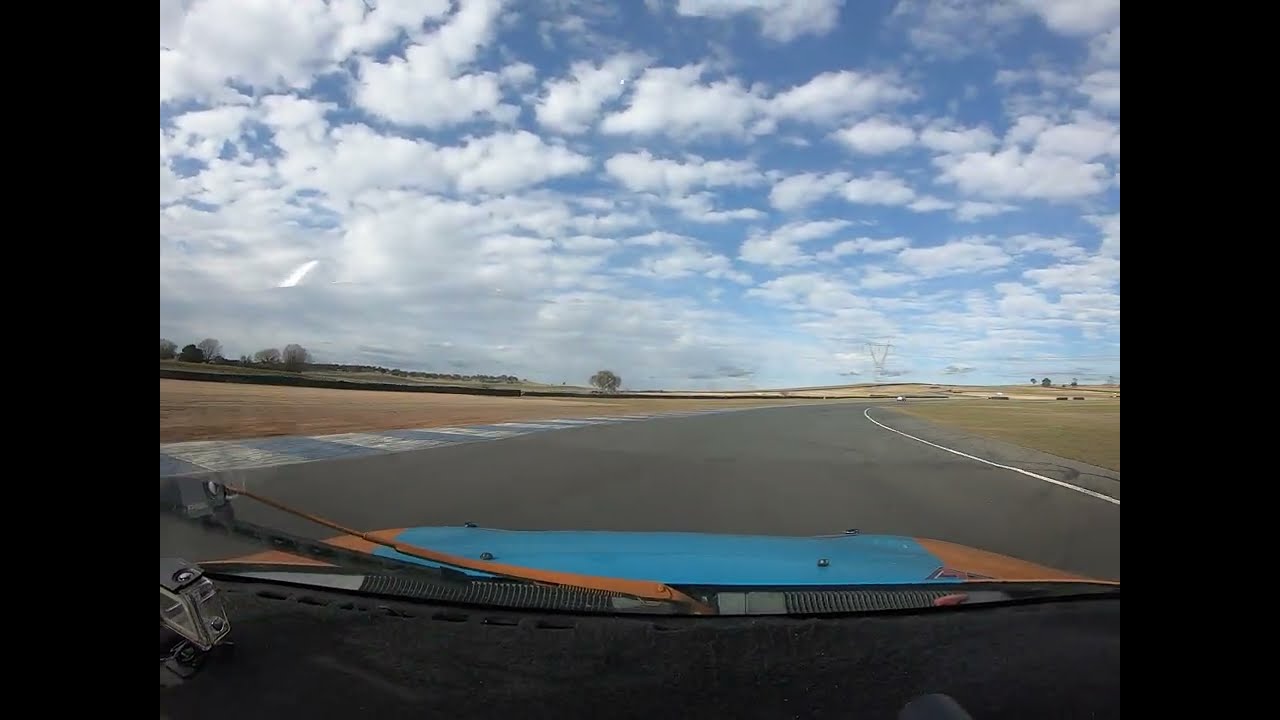This photograph, taken from inside a vehicle, appears to capture the view out the front windshield, likely from a dash cam perspective. Dominating the foreground is the hood of the car, prominently featuring a blue center and orange sides. The roadway ahead is a deserted, single-lane path, potentially a racetrack or test road, curving off to the right in the distance. The road is bordered on the left by alternating white and black squares, with a white line demarcating the edge. Surrounding the road is a landscape of brown dirt or short grass, devoid of greenery. The scene is characterized by a flat, open expanse with a few low rises in elevation and a distant power line. The sky occupies a substantial portion of the image, showcasing a vivid blue canvas dotted with numerous puffy white clouds. Overall, the image depicts a serene yet dynamic setting, emphasizing the car's bold colors against the tranquil, expansive backdrop.